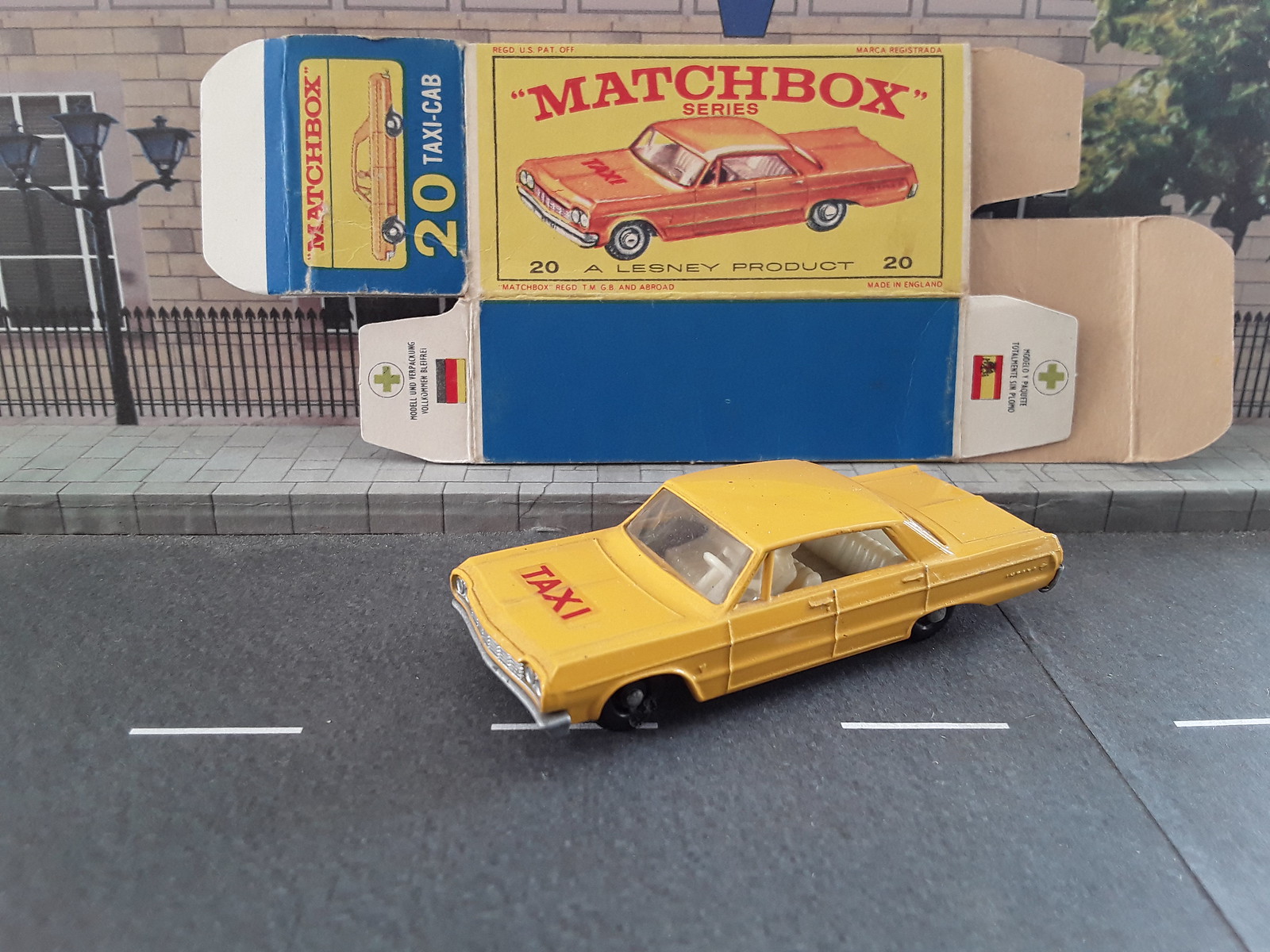The image depicts a detailed scene of a toy Matchbox car set on a small, realistic-looking street corner made out of plastic and cardboard. This yellow car, adorned with red letters spelling "Taxi" on its hood, mimics a classic city taxi. Behind the car sits a slightly worn, vintage Matchbox Series box featuring an illustration of an orange taxi and marked with details such as "20, a Lesney product," with the box itself sporting a blue and yellow color scheme. The setting includes a black picket fence, a lamppost with three lights, a sidewalk with white street lines, and a backdrop suggesting a building with three windows, enhancing the authenticity of the miniature urban scene.